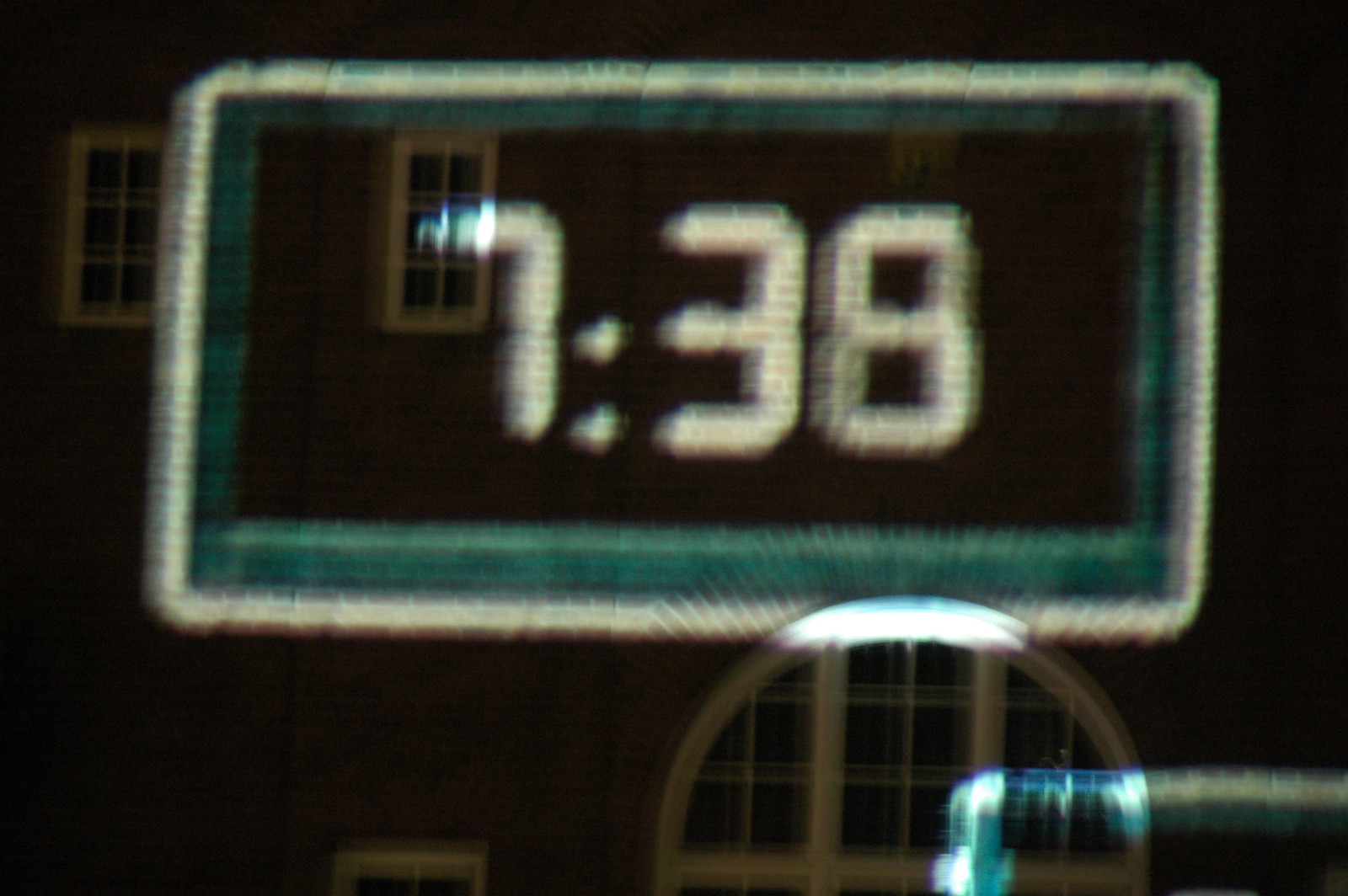This photograph features a highly pixelated, retro-style digital clock displaying the time "7:38" in bright white digits. The clock, projected onto a brick-colored building, is framed by a dark teal rectangle set within a larger white border, evoking an old computer screen's appearance. The building's facade showcases a series of windows, with two smaller, white-framed windows on the upper left and a large, arched window on the lower section. This arched window, reminiscent of church architecture, has three panes across the top and a larger pane below. The background brick structure looks dark brown with a mix of yellowish and tannish shades, suggesting its aged condition. The scene is enriched by subtle reflections on the clock-projection surface, hinting at possible outdoor surroundings, including light blue and black elements in the lower right corner.